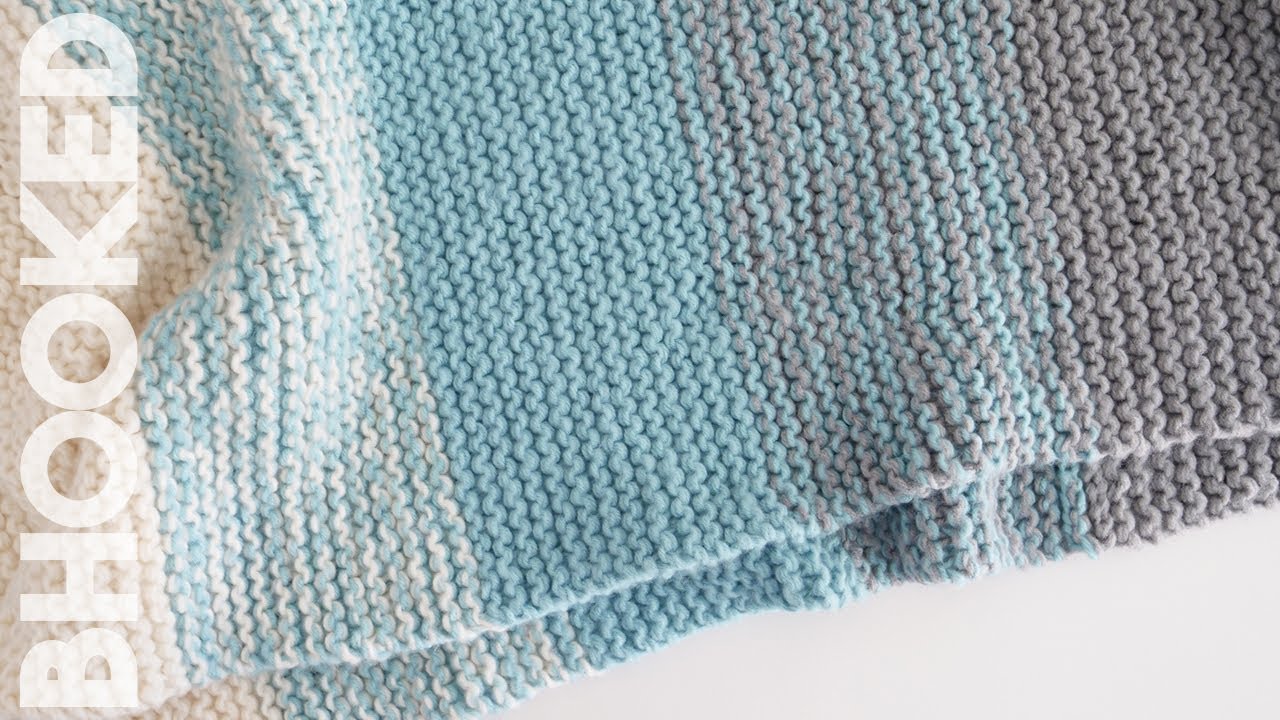This photograph showcases a tightly knitted fabric piece, possibly a scarf, blanket, or tablecloth, set against a white background. The image is zoomed in, revealing the intricate stitching and a variety of colors in a striped pattern. The dominant hues include white, teal, light green, red, peach, grayish purple, cream, and pale blue. Along the left edge of the photo, the text "B-H-O-O-K-E-D" is prominently displayed, suggesting the brand of the stitching. The piece appears handmade and could be featured in an advertisement, web catalog, or for promoting a type of yarn. Despite the close-up view making it hard to definitively identify the item, its vibrant colors and detailed craftsmanship are evident.